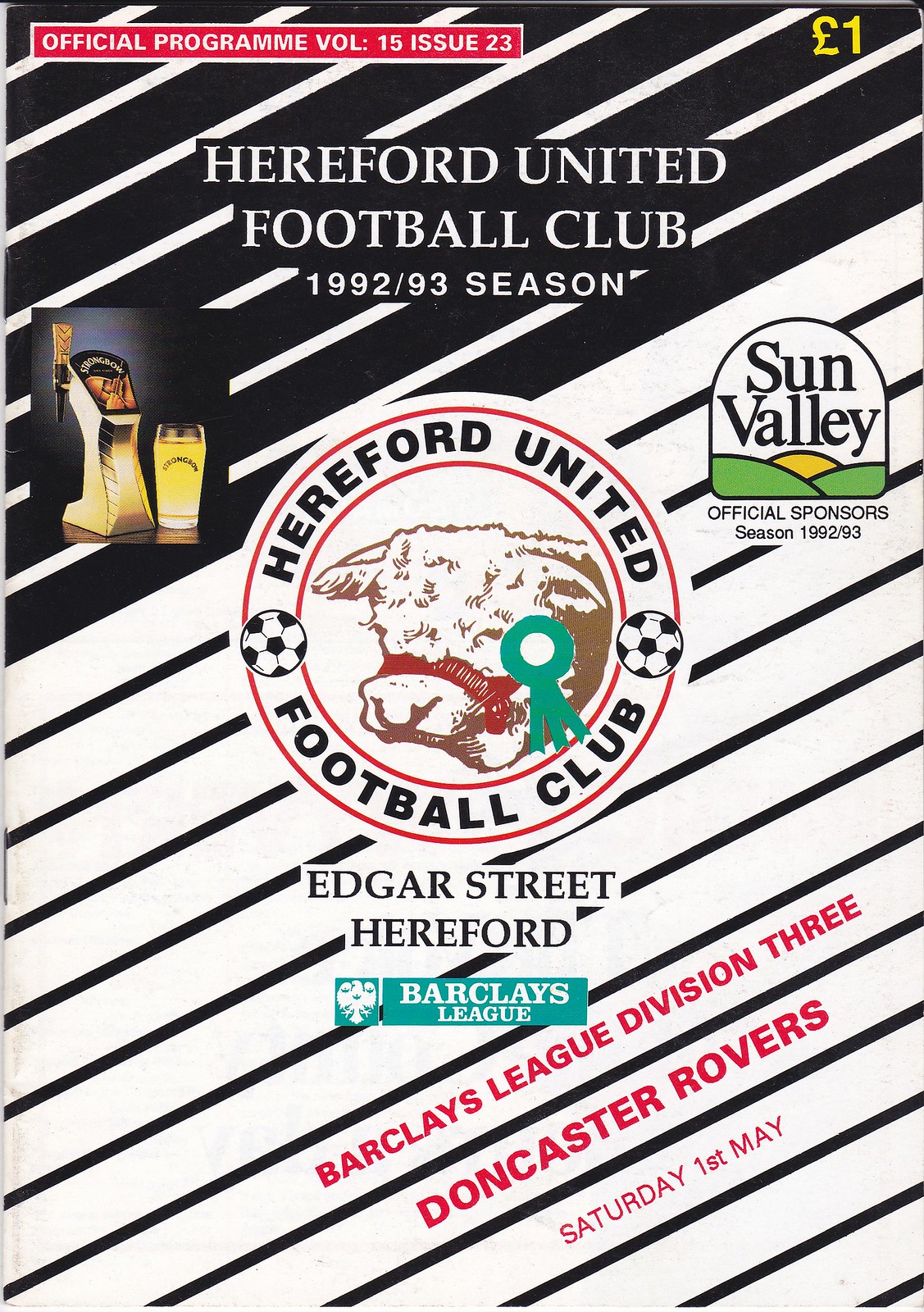This image showcases the front cover of an official program for the Hereford United Football Club, dated for the 1992-1993 season. The cover page, which appears to be black and white with touches of red, features a mix of details including the title "Official Program, Volume 15, Issue 23" prominently displayed in the upper left corner. The cover also lists specific game details: "Barclays League, Division 3, Doncaster Rovers, Saturday, 1st May". In the center, there is a distinct image of a cow adorned with a red halter and a blue ribbon. The backdrop includes various logos and advertisements, such as the Sun Valley Official Sponsor logo in the upper right corner. The bottom part contains text indicating the location, "Edgar Street, Hereford," and "Hereford United Football Club." This setting suggests that the program, likely priced at one British Pound, is a collectible item given out to fans attending a soccer game. The colors present in the image are a mix of white, black, gray, red, yellow, orange, green, and maroon, giving it a vivid yet vintage appearance.